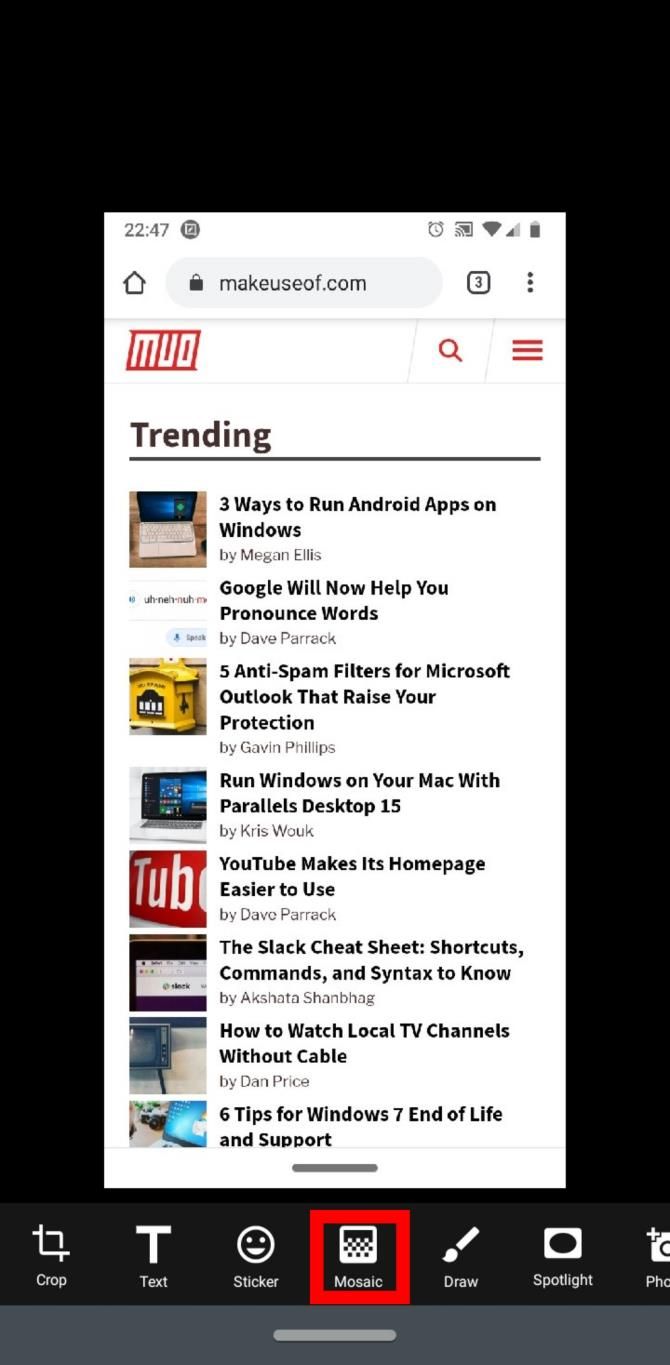The screenshot captured is of the "MakeUseOf" website, identified by the "makeuseof.com" text at the top in black letters. There's a home icon indicating three open tabs and three black dots in the upper part of the screen. Below this, encased in a red outline, are the letters "MUO" (MakeUseOf's acronym) in white.

Adjacent to the logo is a white search bar with a red magnifying glass icon and additional red lines symbolizing other options. Beneath the header, the word "Trending" is prominently displayed in bold black letters with a black line under it. Following this are a series of article titles accompanied by corresponding images:

- **Three Ways to Run Android Apps on Windows**
- **Google Will Now Help You Pronounce Words**
- **Five Anti-Spam Filters for Microsoft Outlook That Raise Your Protection**
- **Run Windows on Your Mac with Parallels Desktop 15**
- **YouTube Makes Its Home Page Easier to Use**
- **The Slack Cheat Sheet: Shortcuts, Commands, and Syntax to Know**
- **How to Watch Local TV Channels Without Cable**
- **Six Tips for Windows 7 End of Life and Support**

At the bottom, editing options for the screenshot are visible, each with both an icon and corresponding label in white text. The options are:
- **Crop** (highlighted by both a word and icon)
- **Text**
- **Sticker**
- **Mosaic** (marked with a thick red square border)
- **Draw**
- **Spotlight**
- **Photo**

These tools are likely part of a screenshot editing toolbar.